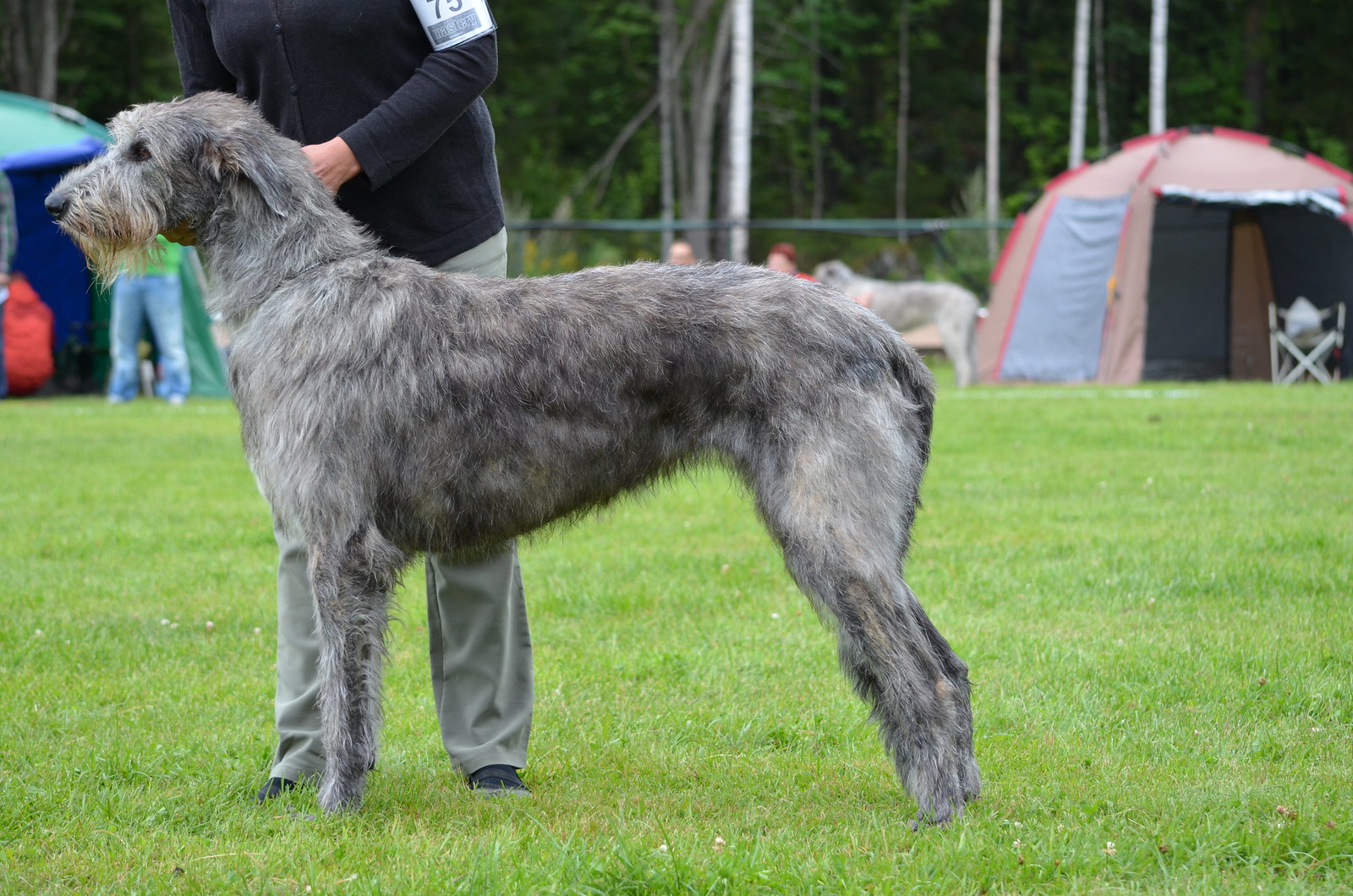This full-color photograph captures an outdoor scene on an overcast day, with a subdued daytime light. In the background, a dense line of trees is partially obscured by several white flagpoles and a chain-link fence. Scattered along the fence line, there are camping tents, with one folding chair visible and a pair of blue-jeaned legs hinting at another person’s presence. The main focus of the image is a dog handler and her grey Irish wolfhound, possibly participating in a dog show, as suggested by the handler’s number 75 tag on her sleeve. The handler, clad in a dark cardigan and khaki pants, appears to be adjusting the dog’s collar. The tall, wiry-coated dog has a brownish-grey hue, with distinctively browner fur around its mouth, standing almost chest-high to the handler. Other tents in the background hint at the presence of more dogs and participants, creating a lively yet serene atmosphere.